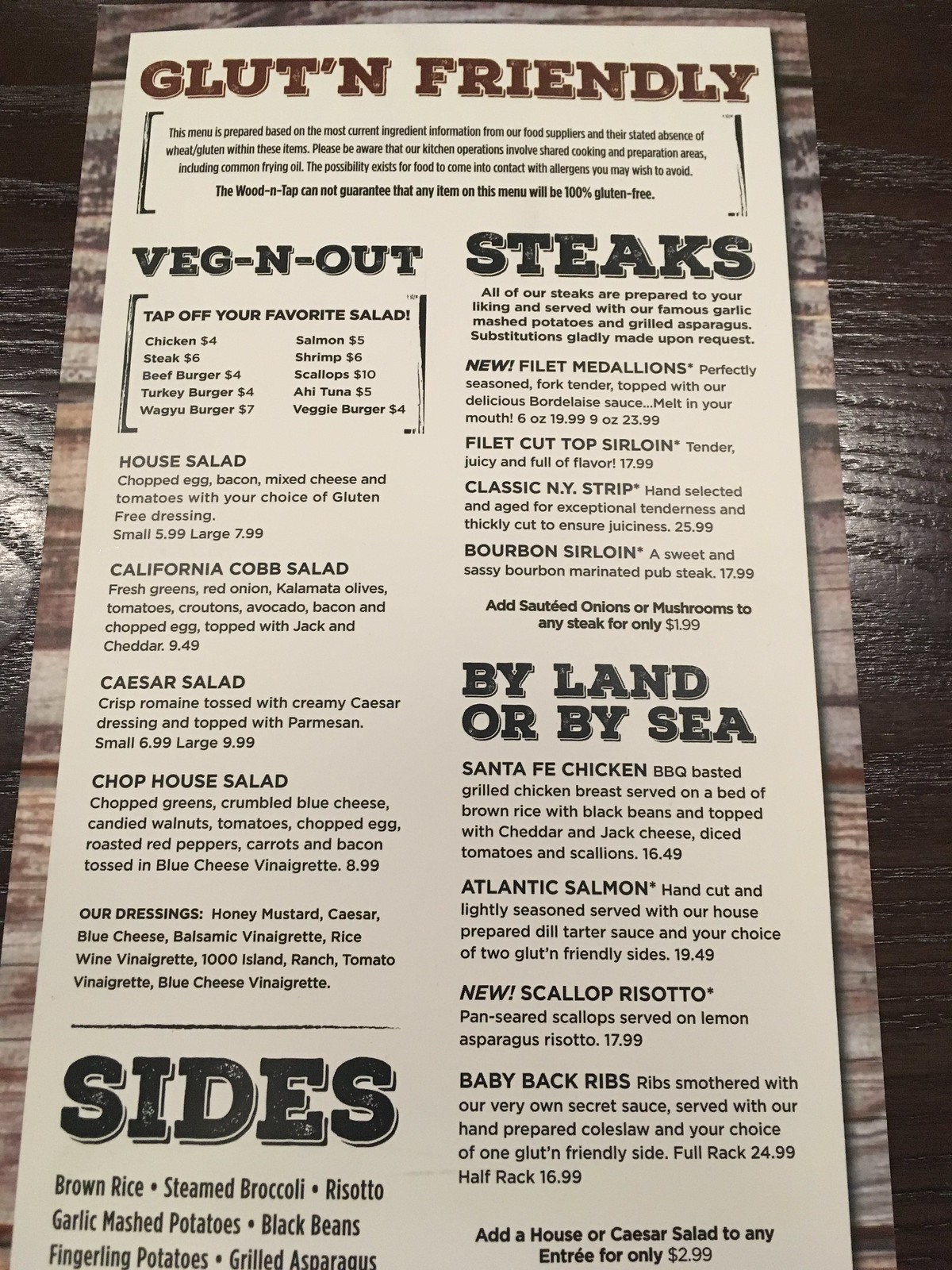This image portrays a meticulously detailed menu set against a beige backdrop, adorned with text in various sections. At the top of the menu, the phrase "GLUTEN-FRIENDLY" is prominently displayed in bold red capital letters. It’s noticeable that the word "GLUTEN" includes an apostrophe. The menu provides a disclaimer that it is prepared using current ingredient information from suppliers and mentions that, despite the absence of wheat gluten in certain items, the shared kitchen environment, including common frying oil, cannot entirely prevent allergen cross-contact. The establishment, "The Wood and Tap," thus emphasizes that no menu item can be guaranteed to be 100% gluten-free.

Beneath this disclaimer is the heading "VEG and OUT," followed by a section dedicated to various steak options. Highlights include:
- **Filet Medallions**: 6 ounces for $19.99, perfectly seasoned, fork-tender, and topped with a delicious bordelaise sauce.
- **Filet Cut Sirloin**: Tender, juicy, full of flavor for $17.99.
- **Classic NY Strip**: Hand-selected, aged for tenderness, thickly cut for juiciness at $25.99.
- **Bourbon Sirloin**: A sweet and sassy bourbon-marinated pub steak for $17.99.
  - Additional toppings like sautéed onions or mushrooms can be added to any steak for just $1.99.

In the right column under the heading "By Land or Sea," the menu offers:
- **Santa Fe Chicken**: Barbecue-basted grilled chicken breast on a bed of brown rice with black beans, topped with cheddar, jack cheese, diced tomatoes, and scallions, priced at $16.49.
- **Atlantic Salmon**: Hand-cut, lightly seasoned, served with house-prepared dill tartar sauce and two gluten-friendly sides at $19.49.
- **New Scallop Risotto**: Pan-seared scallops on lemon asparagus risotto for $17.99.
- **Baby Back Ribs**: Ribs smothered in a secret sauce, served with hand-prepared coleslaw and a gluten-free side, priced at $4.99.

An addition of a house or Caesar salad to any entrée is available for $2.99.

On the left, under the heading "Veg In and Out," the menu lists customizable salads and proteins including:
- **Chicken**: $4.00
- **Salmon**: $5.00
- **Steak**: $6.00
- **Beef Burger**: $4.00
- **Turkey Burger**: $4.00
- **Wagyu Burger**: $7.00
- **Shrimp**: $6.00
- **Scallops**: $10.00
- **Ahi Tuna**: $5.00
- **Veggie Burger**: $4.00

Salad options feature:
- **House Salad**: With chopped egg, bacon, mixed cheese, and tomatoes, offered in small for $5.99 and large for $7.99.
- **California Cobb Salad**: Fresh greens with red onion, kalamata olives, tomatoes, croutons, avocado, bacon, chopped egg, topped with jack and cheddar for $9.49.
- **Caesar Salad**: Crisp romaine tossed in creamy Caesar dressing, topped with parmesan in small for $6.99 and large for $9.99.
- **Chopped House Salad**: Featuring greens, blue cheese, candied walnuts, tomatoes, chopped egg, roasted red peppers, carrots, and bacon in blue cheese vinaigrette for $8.99.

Dressings include options like honey mustard, Caesar, blue cheese, balsamic vinegar, rice wine vinaigrette, Thousand Island, ranch, and tomato vinaigrette.

Sides available are brown rice, steamed broccoli, risotto, garlic mashed potatoes, black beans, fingerling potatoes, and grilled asparagus.